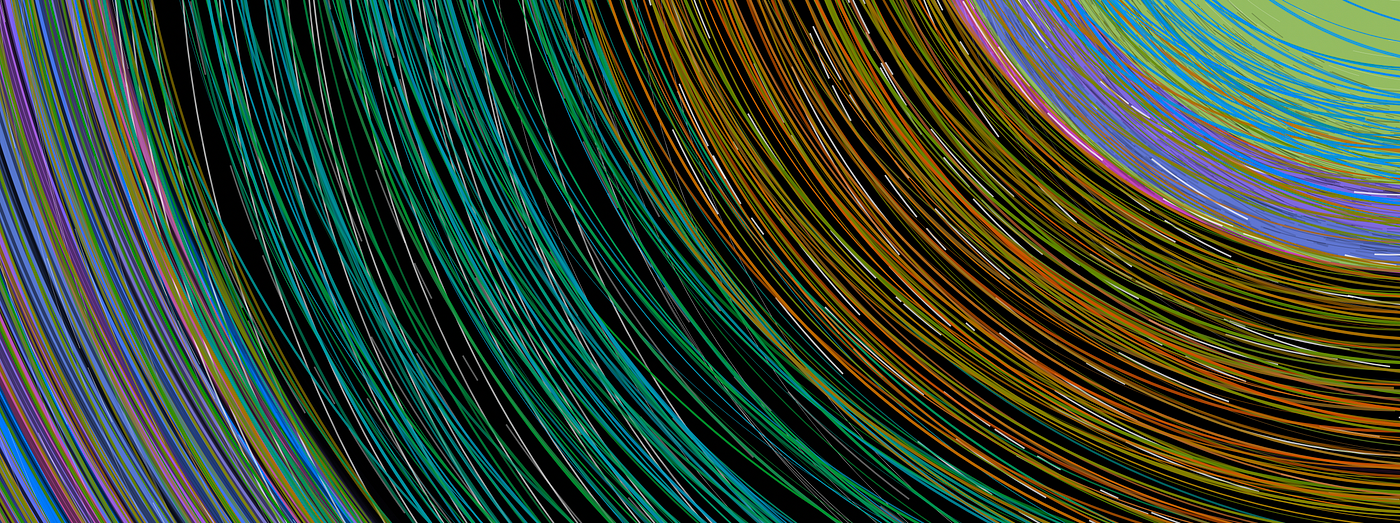This vibrant color photograph presents an abstract, artistic depiction, closely resembling either a detailed painting or a close-up of thin, intertwined cables. The horizontal, rectangular image showcases an intricate pattern of very thin concentric circles and arched lines, generating a rich tapestry of colors. Dominating the composition, lime green, blue, purple, and various earth tones like browns create a visually engaging sequence that seamlessly transitions into different hues, including pinks and reds. The top right corner starts with lime green and baby blue, then introduces oranges and purples; the background darkens with blacks interspersed with orange, green, red, and hints of white. Towards the left, the colors evolve into vibrant greens and blues, culminating in purples at the bottom left. The lines, as fine as wires, form a mesmerizing, almost solar-system-like appearance, suggesting a time-lapse of orbiting space debris. The cropped image focuses on a portion of this intricate circular and linear pattern, enhancing its abstract, snapshot-like quality devoid of any text, emphasizing the colorful symphony of meticulously arranged lines.